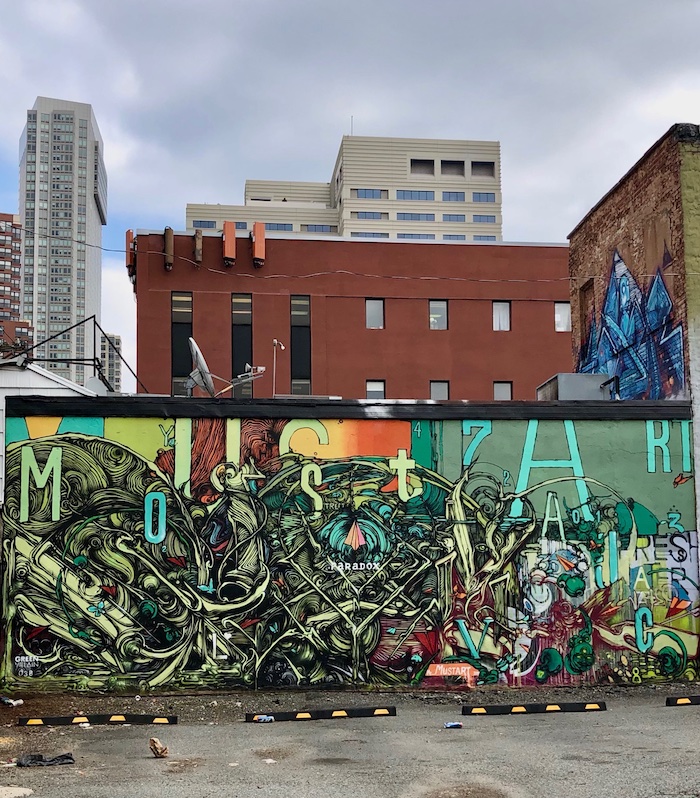In this intricate urban photograph, the scene is divided almost symmetrically by the roof of a grafitti-covered building situated in the foreground, in what appears to be a parking lot with black and yellow car bump stoppers. The wall of the building is a canvas for highly detailed and colorful graffiti, featuring a medley of letters, numbers, and vibrant patterns dominated by dark green circles with shades of yellow, white, red, and peach. There are letters like M, O, S, T, C, U, 7, A, among others, in various colors, creating a visually chaotic yet artistic display.

To the right, an older, worn brown building adorned with large blue graffiti adds to the urban tapestry. Rising behind this edifice is a smooth, rust-colored modern building. Further back, a creamy beige or white building features horizontally ridged siding and small, rectangular windows that resemble bar graphs. Dominating the far left of the background is a tall, creamy white skyscraper, while another rust-colored skyscraper stands further to the left. A satellite dish and other utility installations can also be seen atop the graffiti-covered building. All these structures are set against a cloudy sky, adding a muted tone to the otherwise color-rich scene.